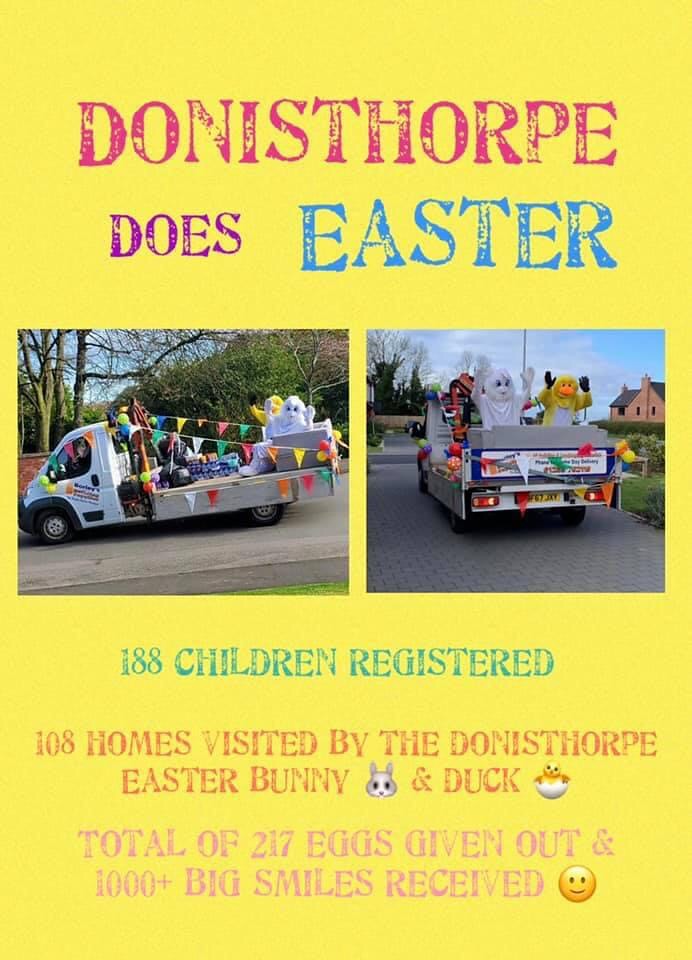This is a vertically oriented, rectangular poster set on a solid yellow background. At the top, in somewhat faded red letters, it reads "Donisthorpe Does Easter." Below this heading, in faded purple and blue lettering, the words "Does Easter" are reiterated. The central portion of the poster features two square images of a float; one shows a left-side view of the float on a road, and the other depicts the back-side view on what appears to be a brick walkway. Both images highlight a flatbed truck adorned with decorations, carrying people dressed in large bunny and chick costumes, waving to an unseen crowd.

In the float photographs, a banner is visible but its text is unreadable. Underneath these pictures, the green text states, "188 children registered," followed by "108 homes visited by the Donisthorpe Easter Bunny" in similar text. Additionally, there are small images of a bunny and a duck, as well as a chick and an egg. The poster concludes with light purple text saying, "A total of 217 eggs given out and 1,000+ big smiles received," accompanied by a smiley face. The poster also features a splash of various colors, including yellow, purple, blue, red, green, and light purple.